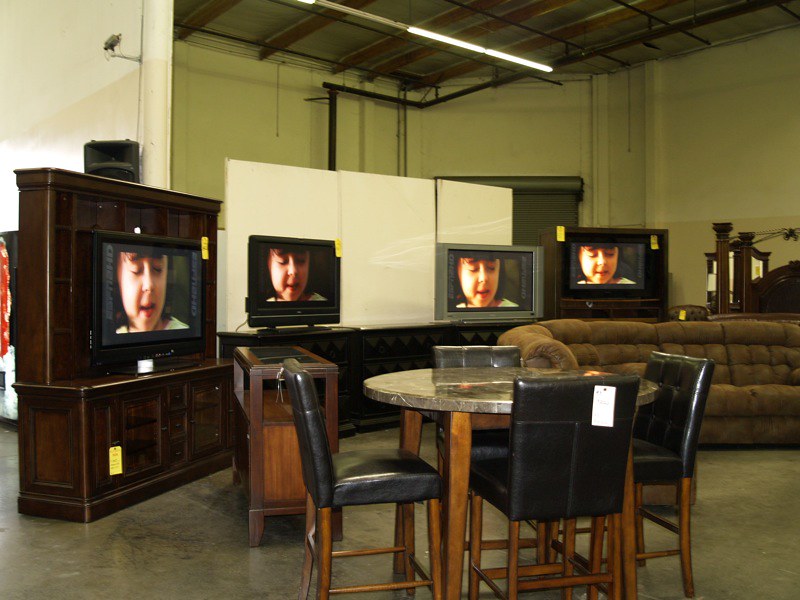This image captures a detailed scene from a furniture showroom bathed in a slightly yellow tint under an industrial open roof with exposed black piping and track lighting. The walls are cream-colored with off-white sections and three white panels behind the furniture.

In the center of the image is a round dining table with a gray marble top and reddish-brown wooden legs. Surrounding the table are four chairs with black faux leather upholstery and matching wooden legs. Positioned in the background to the right is a large, cushiony brown sectional sofa.

Prominently displayed along the back wall are two tall wooden media entertainment centers with drawers underneath. They are supporting four flat-screen televisions, arranged in a semi-circle; three are black, while the third one has a gray casing. All the televisions are displaying the same image of a little girl with her eyes closed, and each has a yellow price tag, although the amounts are not legible. Positioned in front of these entertainment units are smaller white boards without backing.

The gray polished concrete floor adds to the industrial ambiance of the space, hinting at a polished, contemporary display in what could be a high-end furniture store. Additional details like paper tags on various items reinforce the showroom setting, showcasing a mix of stylish and comfortable furniture pieces for potential buyers.